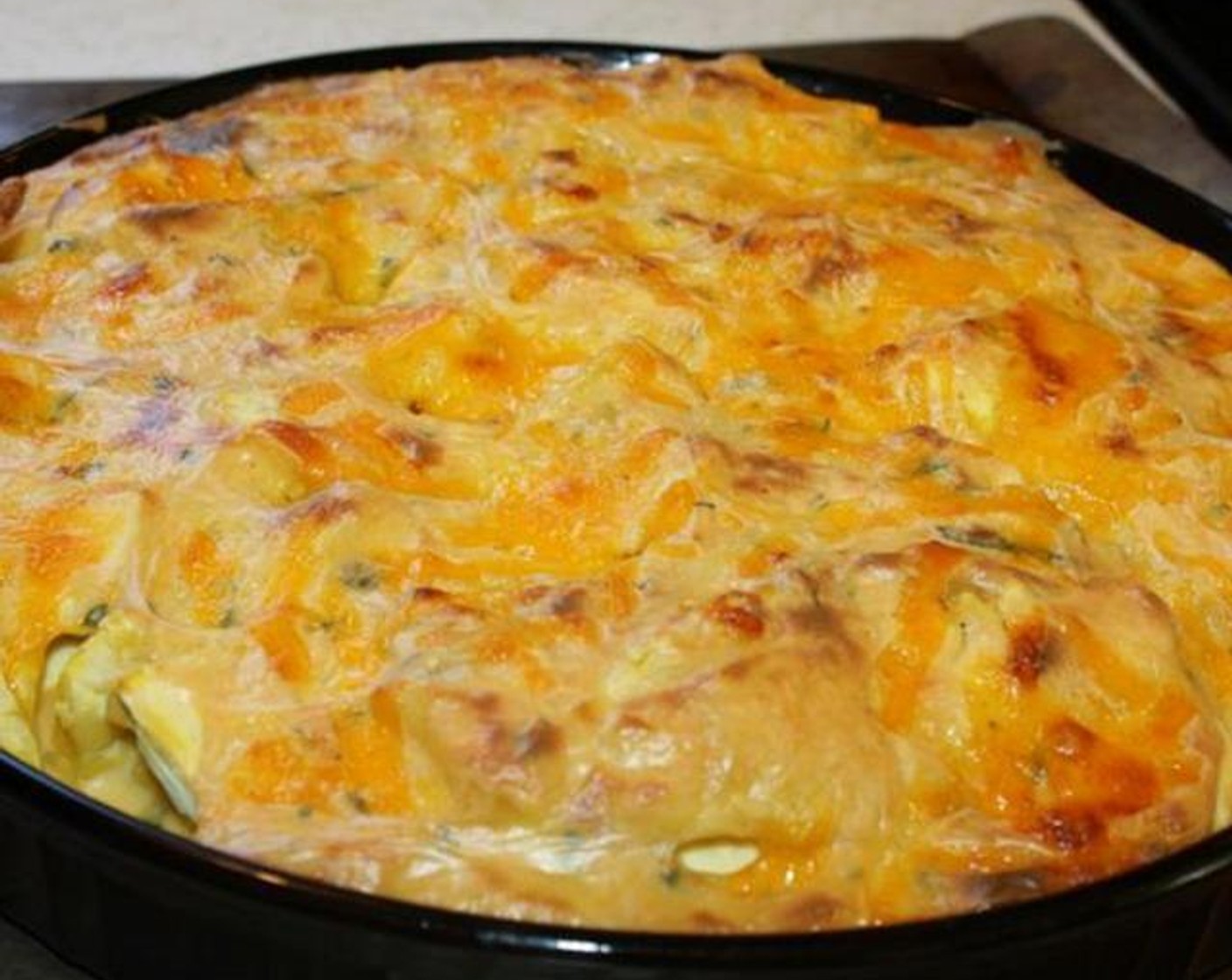In the image, we see a freshly-baked casserole nestled in a round, black cast-iron skillet. The golden top layer suggests it might have been broiled, showcasing a spectrum of colors from yellow to orange and brown. The cheese on top appears gooey and inviting, hinting at the dish's rich, cheesy flavor that possibly includes a mix of cheese and egg. Vegetables and possibly meat peek through the surface, indicating a hearty blend of layers within. The skillet also has a piece of foil, likely used to keep the ingredients from sticking. The dish appears glistening, with a slight shine, emphasizing its just-out-of-the-oven warmth and melt-in-your-mouth appeal. The background subtly features a platform, complementing this detailed snapshot of a sumptuous brunch casserole.